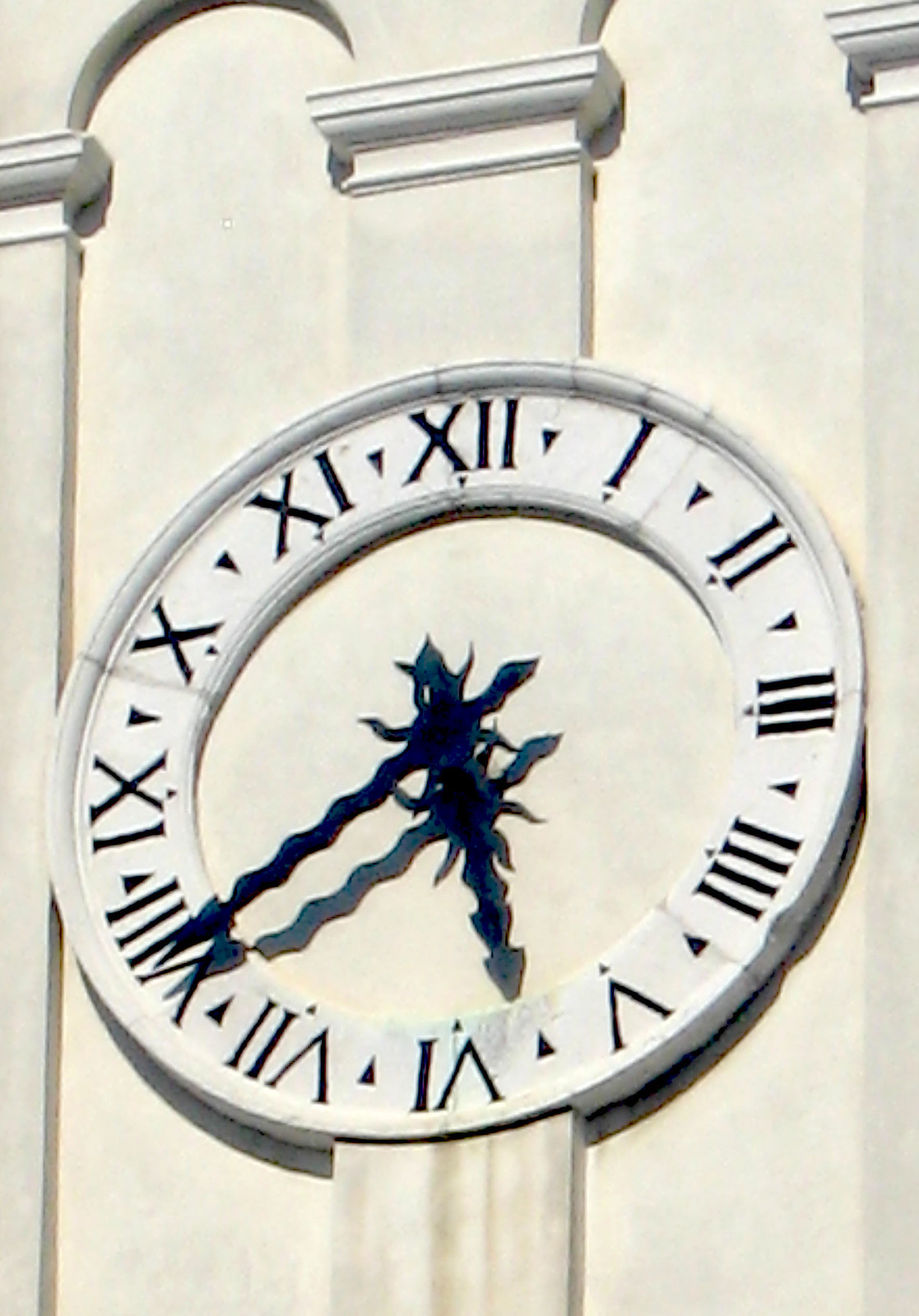An image depicting an outdoor clock mounted on a white stone or brick wall, bathed in bright sunshine. The sunlight, emanating from above and slightly to the left of the clock, illuminates the scene with a stark clarity. The building's façade features sections with raised columns that create a rhythmic pattern of vertical lines. These columns are interspersed with arched tops, each capped with a detailed plinth, creating a classic architectural aesthetic reminiscent of a colonnade with filled gaps.

The clock itself is a round, likely stone or marble structure, seamlessly integrated into the wall's design. Its face features a ring of white set against the cream-colored building, devoid of any column detail interrupting the center. Encircling the clock, black-painted Roman numerals mark the hours, contributing to its elegant appearance. The hour and minute hands, crafted from wavy black iron, indicate the time is approximately 5:40. The combination of the intricate architectural elements and the classic design of the clock creates a timeless and harmonious visual appeal.